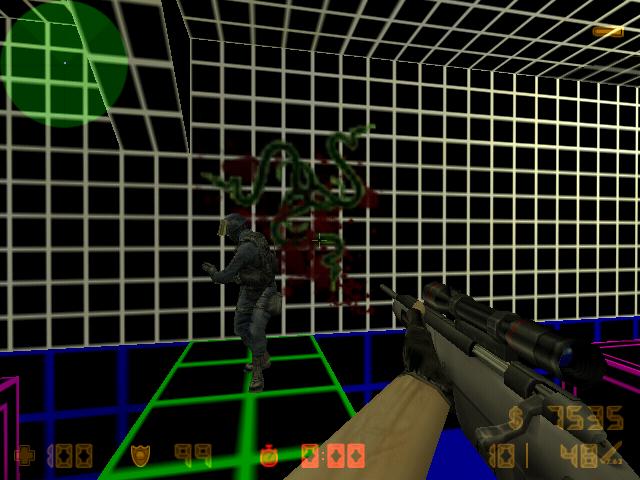This image is a screenshot from a first-person shooter video game, where the perspective is that of a soldier wearing black gloves with his thumb sticking out. The soldier, with a fair complexion visible on his left forearm, is gripping a gray sniper rifle, featuring a long black scope and a black barrel. The environment is a dimly lit room with a grid pattern, composed of black squares framed by white lines on the walls and green lines on the floor. To the soldier's front, there is an armored enemy standing on a green grid square, clad in black and gray gear, including brown boots, a helmet, and a bulletproof vest, with a bandolier across his chest. Above the enemy, a snake-like symbol or green snake graphics are visible. The bottom of the screen displays various statistics, such as a health symbol showing 100, a shield symbol at 99, a 000 time symbol, and a monetary value, as well as a score indicating the player's status in the game.